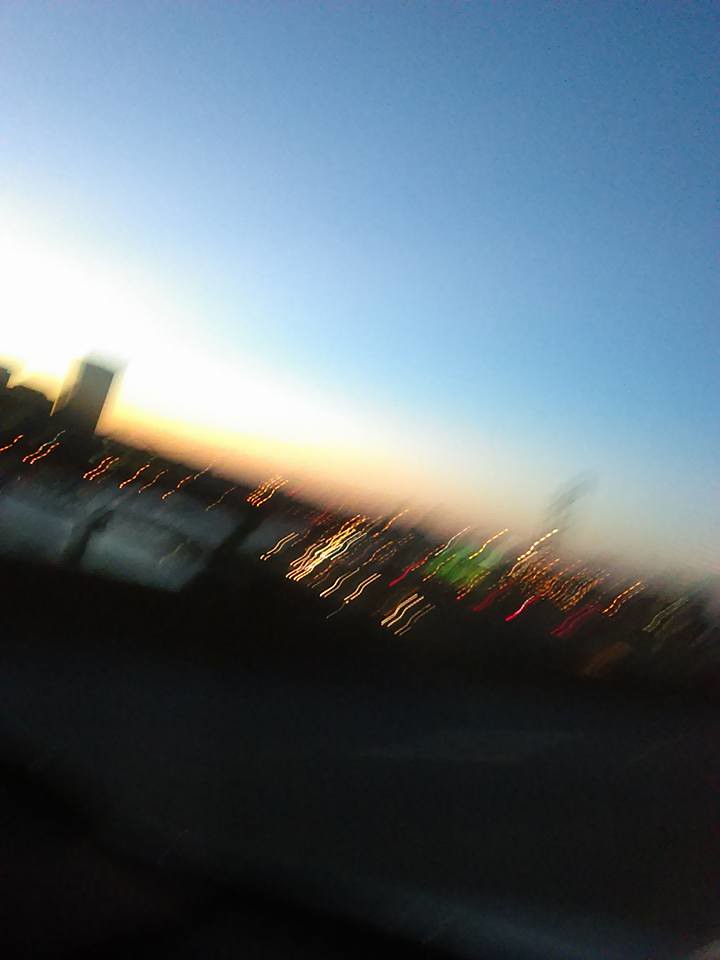This is an abstract depiction captured from inside a moving vehicle at night. The lower third of the image is dominated by a gray section, likely representing the bottom part of a window, adding to the sense of movement. On the left side, there appears to be a reflection on the glass, enhancing the blurred effect. The sky above is a deep blue, transitioning into streaks of white, yellow, and peach hues along the horizon, suggesting a cityscape under artificial lighting.

A prominent gray high-rise, rectangular in shape, stands tall on the left-hand side of the photo. The scene is interspersed with scattered, white, dot-like squiggles that trail upward, creating a dotted path due to the vehicle's motion. These points of light form in clusters, particularly below the horizon and repeated further up.

Different colored squiggles add to the image's vibrancy—greens, pinks, and yellows blend and blur together, giving the scene a dynamic and transient feel, painting an impressionistic portrayal of city lights and their reflections.